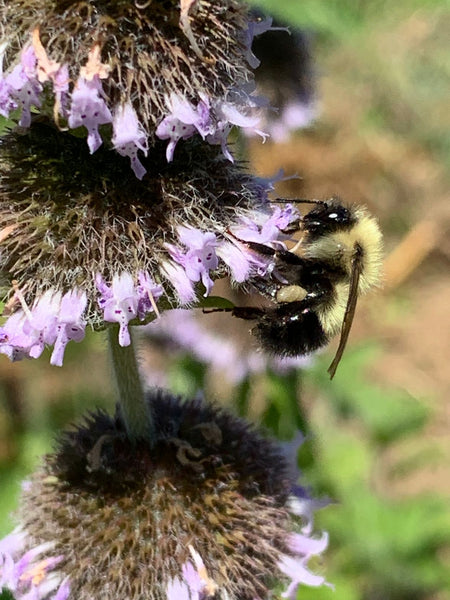The image is a color photograph in portrait orientation, capturing a detailed close-up of a yellow and black bumblebee perched on a flowering plant. The bumblebee, with its fur-like structure, is centrally positioned in the image, facing upward with its back toward the right side, and its legs firmly grasping the flower. The flower appears to be a dandelion with a stem that is green in color and three distinct tiers of buds stacked on top of each other. Each tier of buds is domed centrally, surrounded by small brown structures with pale lavender white blossoms around the perimeter. The background, which is out of focus, consists of green leafy structures, suggesting either grass or shrubs. The photograph is taken outdoors in broad daylight, exemplifying wildlife or nature photography with no text present in the image.